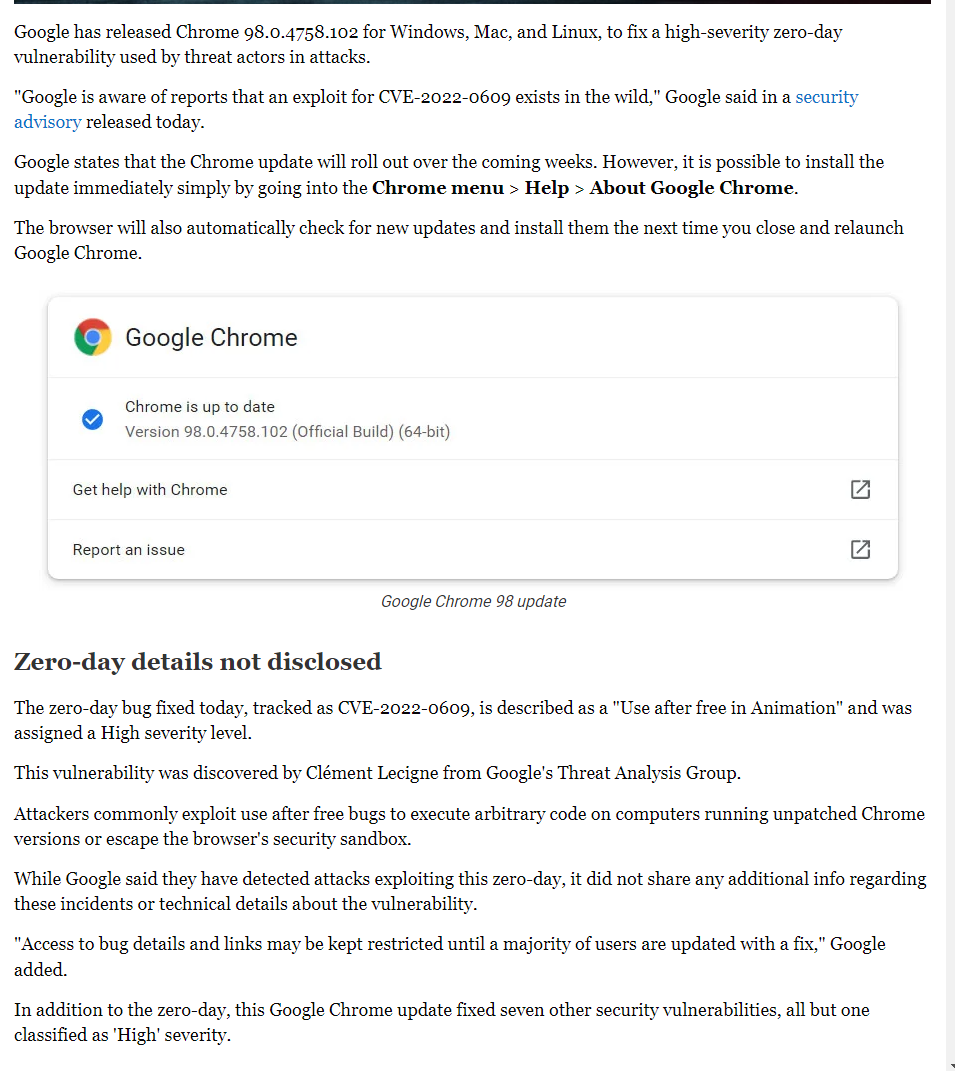**Caption:**

In the midst of an article detailing the recent Google Chrome update, a prominent sub-window takes center stage, showcasing the Google Chrome logo. Below the logo, a blue circle with a checkmark confirms that Chrome is up to date with version 98.0.4758.102. The sub-window provides two interactive options: "Get help with Chrome" and "Report an issue," both as clickable links. The surrounding article elaborates on Chrome's release version 98.0.4758.102 for Windows, Mac, and Linux, addressing a high-severity zero-day vulnerability that has been exploited by malicious actors. Spanning the rest of the page, the article dives into further details about the update's significance and its security implications, although the original source of the article remains unspecified.